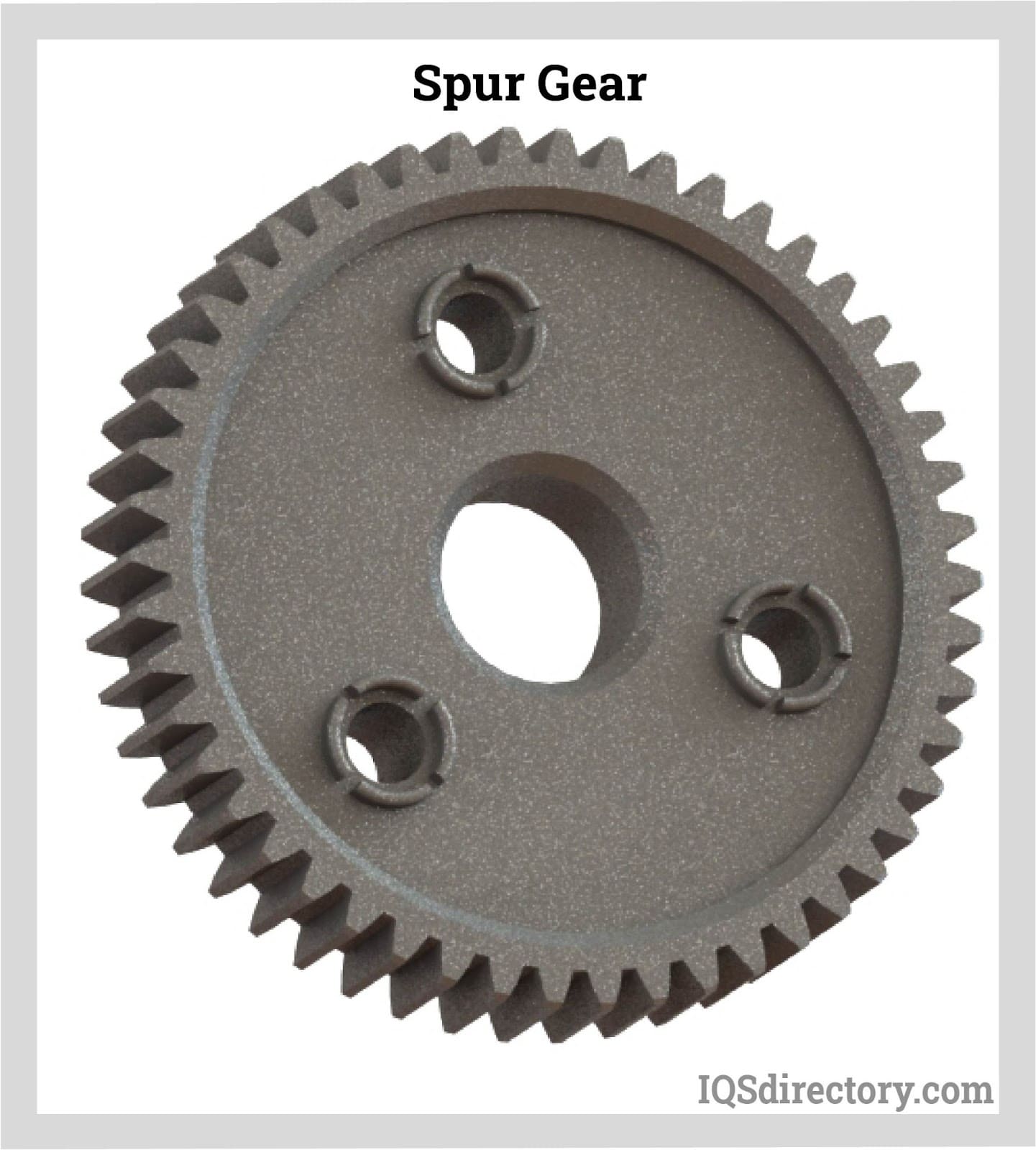The image features a photograph of a gray metal spur gear, prominently displayed against a white background with a light gray border. The gear, slightly taller than it is wide, has numerous teeth lining its circumference, creating a spiky or grooved edge. At the very top, centrally aligned in bold black letters, is the label "Spur Gear." The gear itself is speckled with tiny white spots, adding to its textured appearance.

In the center of the gear is a large circular cutout, designed to accommodate a shaft. Additionally, there are three smaller circular holes equidistant from each other, forming an equilateral triangle when connected. These smaller holes likely serve as points for bolts to secure the gear to a shaft or another component.

In the lower right corner of the image, the URL "iqsdirectory.com" is printed in gray letters, indicating that the image may be sourced from a parts catalog or directory for replacement components. The overall layout is enclosed in a square format, framed by a light gray border, giving the image a clean and structured look.